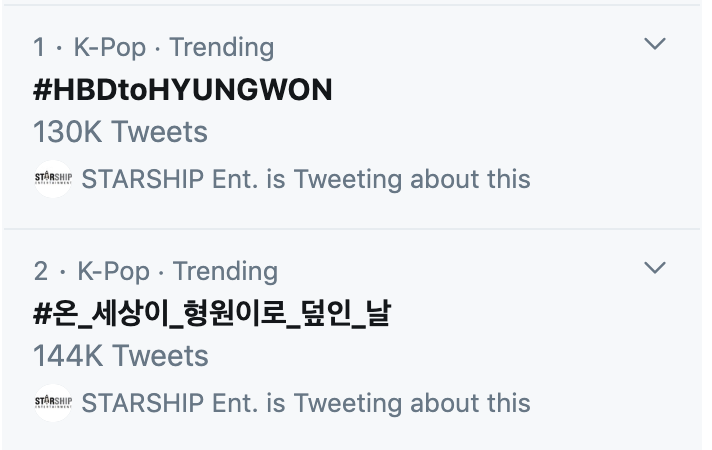Here's a detailed and cleaned descriptive caption for the image:

---

The image appears to be a screenshot from Twitter showcasing trending topics in K-pop. It is divided into two gray rectangles stacked one above the other with a thin gray line separating them.

In the top rectangle:

- **Title**: "No. 1 K-pop Trending"
- **Content**: In bold black text, it displays "HASHTAG HBD to Hyungwon" (spelled as HYUNGWON).
- **Statistics**: Indicates "130K Tweets" in light gray.
- **Source**: Features the Starship Entertainment logo—a white circle with the text "Starship ENT" beside it.
- **User Indicator**: Notes that Starship ENT is tweeting about this trend.
- **UI Element**: There is a small downward-facing arrow icon in the upper right corner.

In the bottom rectangle:

- **Title**: "No. 2 K-pop Trending"
- **Content**: Contains stylized black Asian characters written across the screen.
- **Statistics**: Indicates "144K Tweets" in light gray.
- **Source**: Again, features the Starship Entertainment logo and the text "Starship ENT" beside it.
- **User Indicator**: Notes that Starship ENT is tweeting about this trend as well.
- **UI Element**: A similar downward-facing arrow icon is present in the upper right corner.

---

Feel free to modify any part of this descriptive caption to better suit your needs!